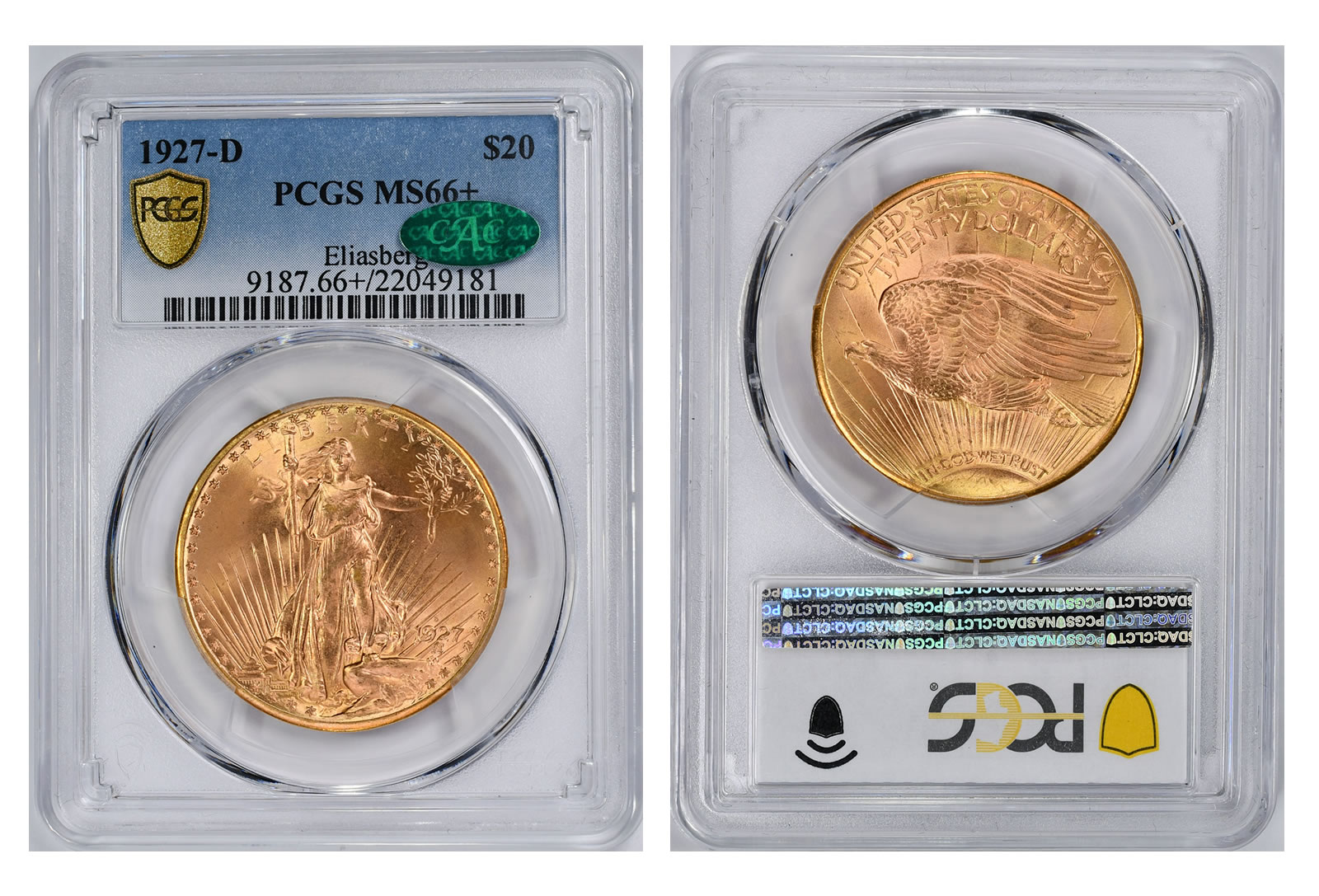The photograph depicts two collectible gold coins encased in a clear protective case. The coin on the left is a 1927 D $20 gold piece, graded PCGS MS 66 Plus. This coin features an image of a woman, presumably Lady Liberty, embracing a man at its center. On the coin on the right, which is the reverse side of the same coin, an eagle faces right with the inscription "United States $20" above it. The case also displays detailed labeling including a serial number, "PCGS MS 66 Plus" grading, and barcode, signifying that it is intended for coin collectors.